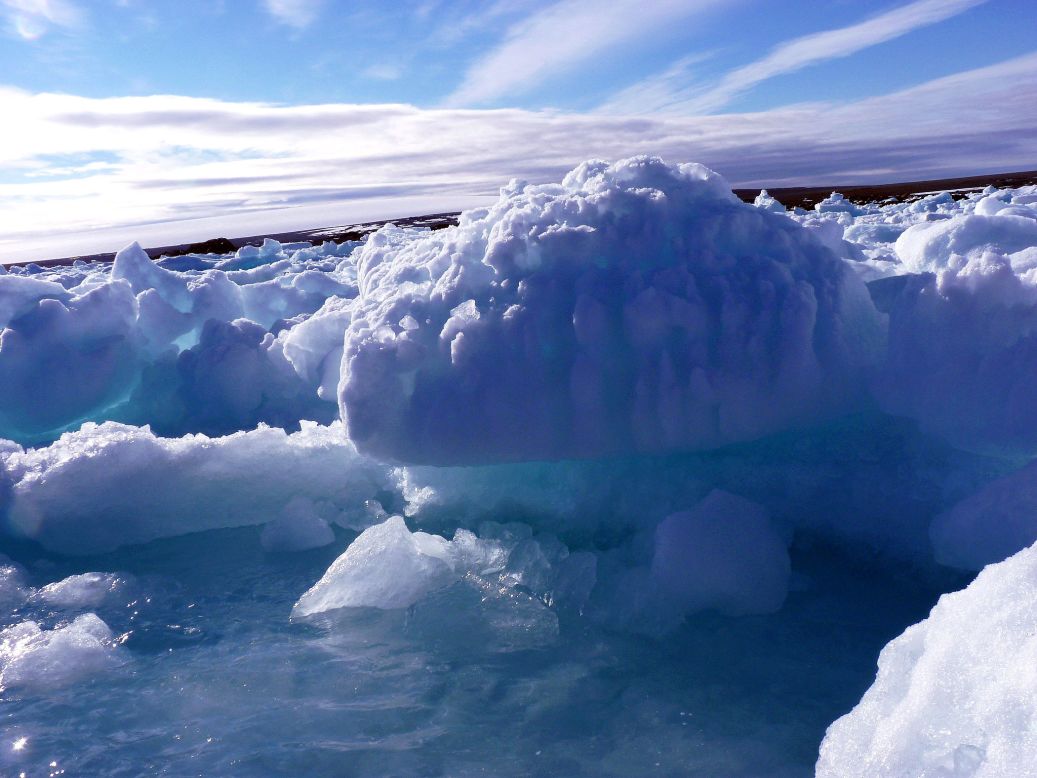This photograph captures a striking scene likely from the Arctic or Antarctic circles, taken during the daytime with sunlight illuminating the area. The landscape is predominantly covered in ice and snow, creating a predominantly white and light blue color palette. The ocean, mostly blanketed in irregular ice formations of varying heights, features one particularly notable dome-like structure in the foreground. Pockets of exposed liquid water disrupt the icy expanse, hinting at the process of melting. Above, the sky is a clear blue dotted with white and gray clouds. The high elevation slopes down towards the horizon, suggesting an ice flow or glacier moving towards the lower-lying ocean. The entire scene is a beautiful yet stark portrayal of a frozen wilderness in transition.